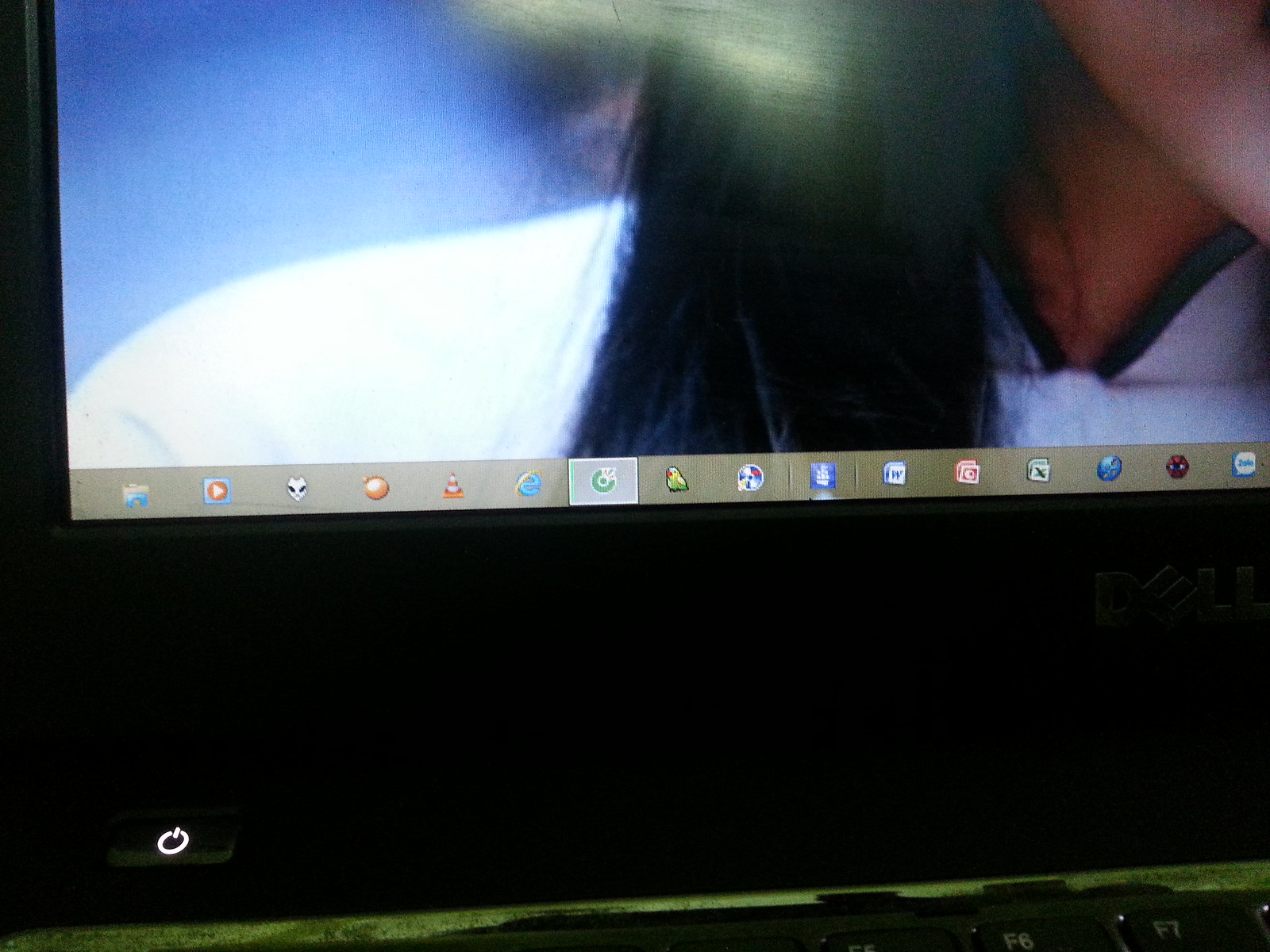The image shows a portion of a computer screen, likely displaying a Windows operating system. The upper part of the image is fuzzy but reveals the lower area of a person's face, noticeable for their jawline and long black hair, which descends to just above their chest. The individual appears to be wearing a white V-neck shirt with a bit of black trim around the neckline. The background behind them is blue, and to the lower right, you can faintly see the 'Dell' logo, suggesting it's a Dell laptop.

At the bottom of the screen, multiple icons are visible, including Internet Explorer, VLC Media Player, and several other unrecognized icons. There's also an orange symbol resembling a skull or alien. A power button with a white light is located on the bottom left, below the monitor. On the bottom right, a small portion of a keyboard can be seen, specifically the F6 and F7 keys. This detailed setup implies a typical computer user interface with various software shortcuts neatly arrayed on the taskbar.